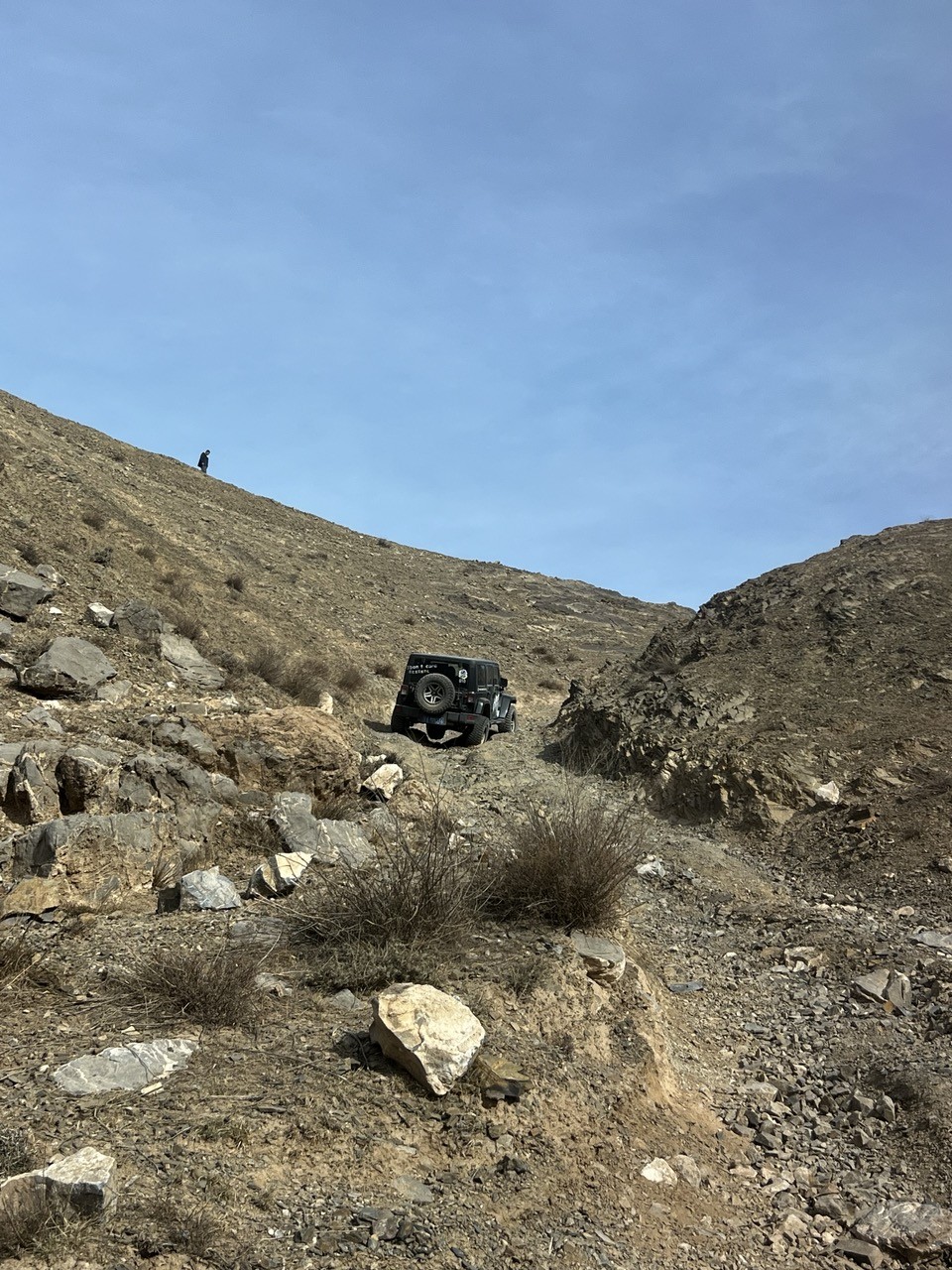Under a perfectly clear blue sky, a rugged dirt road winds its way up a semi-steep mountainside, composed of both small stones and large boulders. Dominating the center of the image is a black Jeep, its spare tire prominently displayed on the back, as it navigates this makeshift path. The dirt road curves upward and around to the right, disappearing into the middle of the picture. In the top left portion of the image, a tiny figure can be seen walking along the edge of the mountain. The left side of the frame is filled with scattered rocks and boulders, stretching from the foreground up to the top of the mountain. The right portion of the image features a rocky hill that extends from the center to the right middle. The foreground is characterized by patches of dry, dead-looking shrubs mixed with dirt and rocks. The bright, wisp-free sky enhances the earthy tones of the scene, accentuating the rugged and raw beauty of this natural setting.